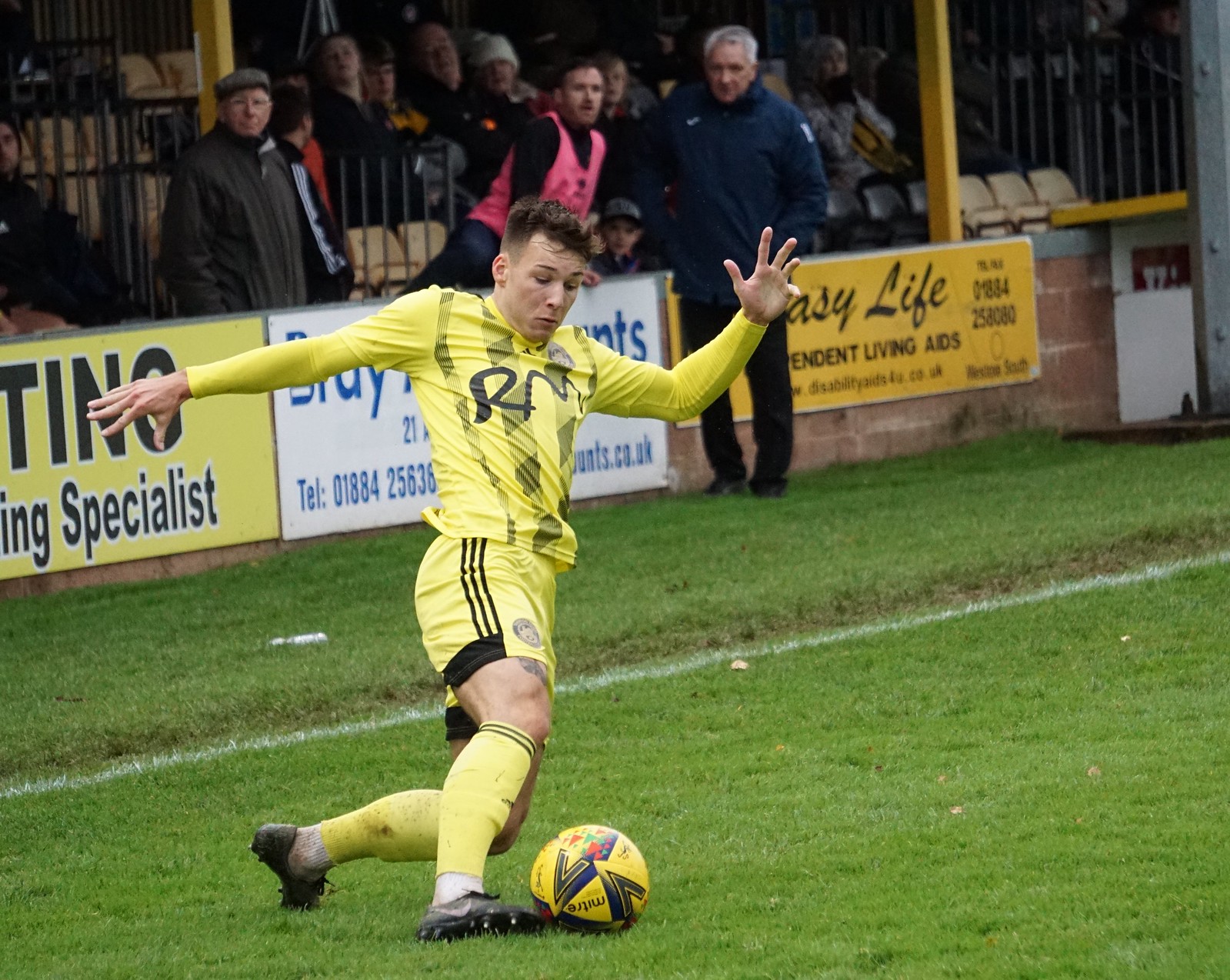In this vibrant, high-definition photograph, a professional soccer player, dressed in a bright yellow uniform complete with cleats, takes center stage on an outdoor soccer field. He is caught mid-action, poised to kick a yellow ball with his right leg extended forward and his back leg bent at a 90-degree angle, toe touching the green turf. His right arm is lifted and bent, while his left arm is extended behind him, and his focused gaze is fixed downward on the ball. The player appears slightly off-balance, showcasing his athleticism and agility. The background reveals a crowded stadium with colorful, enthusiastic fans and a discernable official standing out of bounds on the turf. Minimal yet visible advertisements line the backdrop, partly obscured by the player. The scene is encapsulated with various bright colors, highlighting the dynamic and modern style of the image.